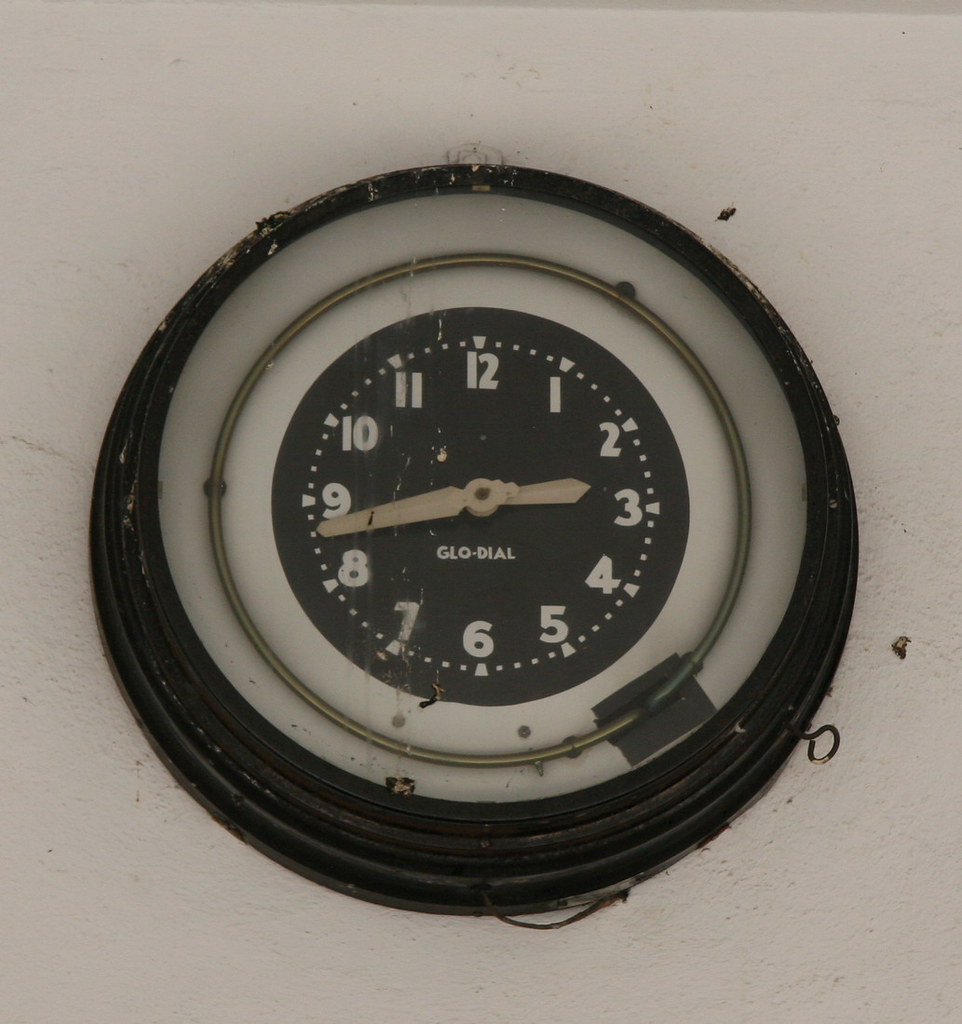The photograph depicts an antique, analog clock with a weathered appearance, hanging on a marked, off-white, possibly drywall surface. The clock features a robust, thick black metal frame showing signs of wear, including rust and white spots, indicative of its age and lack of upkeep. Surrounding the clock face is a set of metal rings, adding to its vintage charm. The clock's face consists of a white outer border and a black central area that houses white numbers and markings. The hands of the clock, colored in light tan, with one long hand and one short hand, indicate the time as 2:43. No second hand is present. The clock bears the label "GLODIAL" in white lettering, right below the hands. Overall, both the clock and the background it hangs on exude an aura of antiquity and disrepair, enhanced by visible stains and markings on the wall.